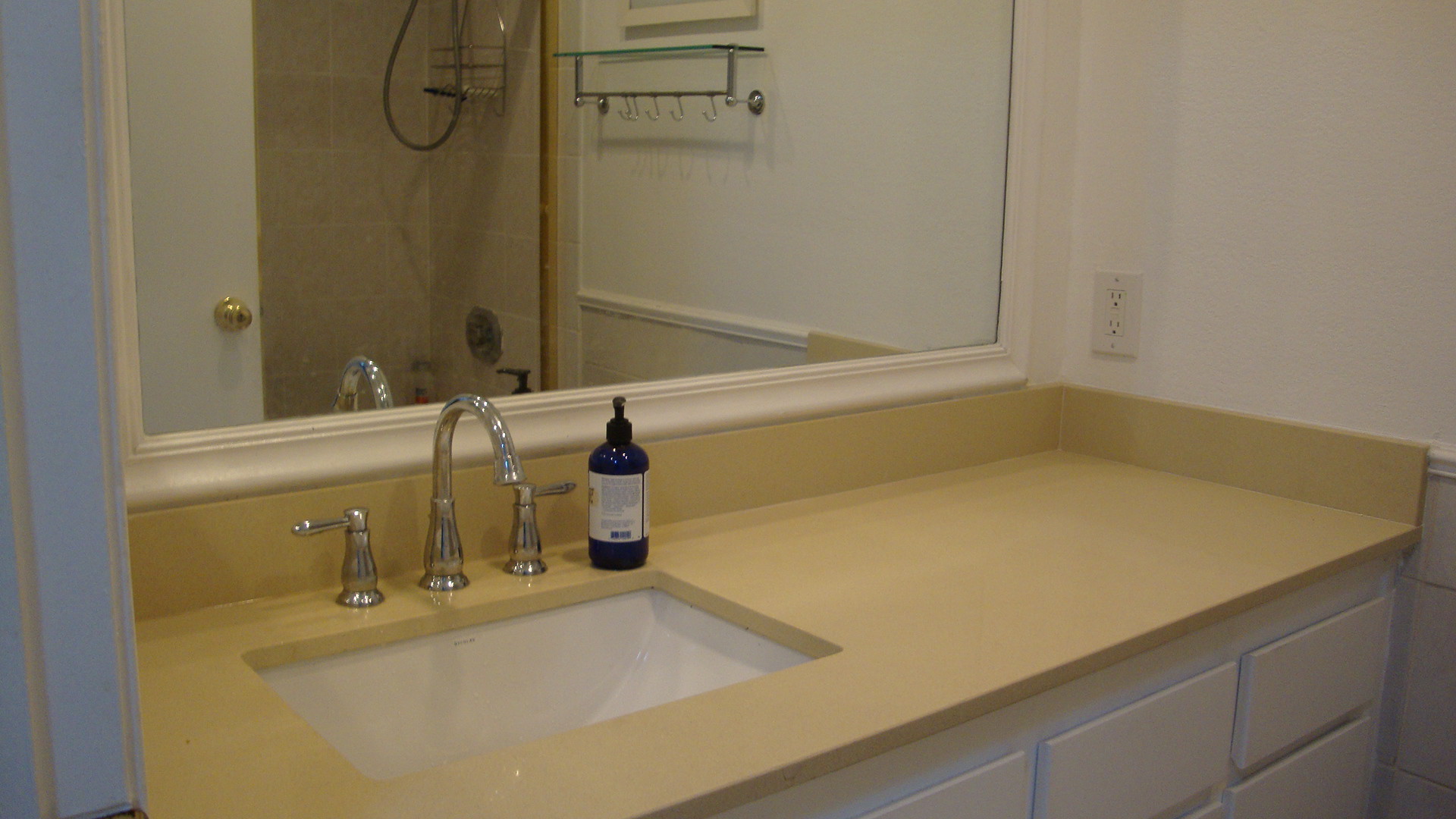This close-up image of a bathroom countertop showcases an off-white wall with an empty electrical outlet plate. The countertop features a rectangular, beige-toned sink with a silver faucet and distinct hot and cold handles. Above it, a large mirror framed in white trim reflects several details: a wooden door with gold knobs, a brown-tiled shower with a hanging shower hose, and a mounted hanger with four hooks on the wall. The scene emphasizes the sink area, capturing the sleek, reflective surfaces and the utilitarian design of this well-appointed bathroom space.